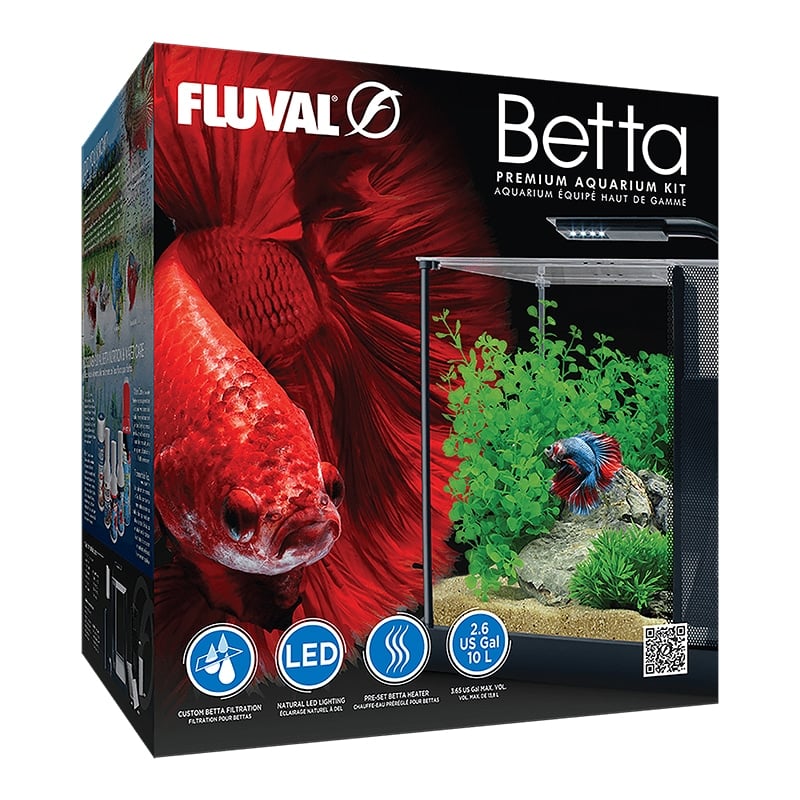This photograph features the packaging for the Fluval Betta Premium Aquarium Kit, prominently displayed with vivid, colorful imagery. In the upper left-hand corner, the brand name "Fluval" is inscribed, while the upper right-hand corner showcases the product name "Betta Premium Aquarium Kit" along with the French translation, "Aquarium Équipe Haute de Gamme." Dominating the left side of the box is a striking image of a red betta fish with flowing, plumage-like fins and bubble eyes set against a dark background. On the opposite side, at the bottom right, is a picture of the aquarium itself, complete with a blue and red betta fish swimming amongst green plants and rocks. The bottom left-hand corner features four circles, each indicating specific product details: one highlights LED lighting, another notes the aquarium's capacity of 2.6 US gallons (10 liters), while the remaining circles depict graphics for "custom betta filtration" and a "preset betta heater."